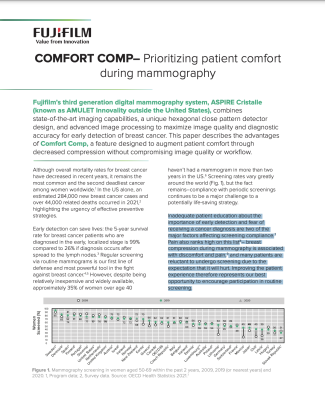The image is an informative pamphlet from Fujifilm, titled "Comfort Comp: Prioritizing Patient Comfort During Mammography." The Fujifilm logo is at the top left corner, with the slogan "Value from Innovation" beneath it. The pamphlet introduces Fujifilm's third-generation digital mammography system, Aspire Cristella, which is known as Amulet Innovality outside of the United States. This system combines state-of-the-art imaging capabilities, a unique hexagonal close pattern detector design, and advanced image processing to maximize image quality and diagnostic accuracy for the early detection of breast cancer. 

The description highlights the Comfort Comp feature, designed to enhance patient comfort by decreasing compression without compromising image quality or workflow. Below the main title and introductory paragraph, there are two columns of smaller text detailing the system's technical specifications and benefits. Towards the bottom right, a paragraph is outlined in blue. 

At the bottom of the pamphlet, there is a gray-background graph indicating some sort of data related to the system's performance, though the specific details and numbers are too small to be legible in the image. The overall layout consists of well-structured text and imagery, but much of the finer print and specific details remain difficult to read due to the small font size and slight blurriness of the image.